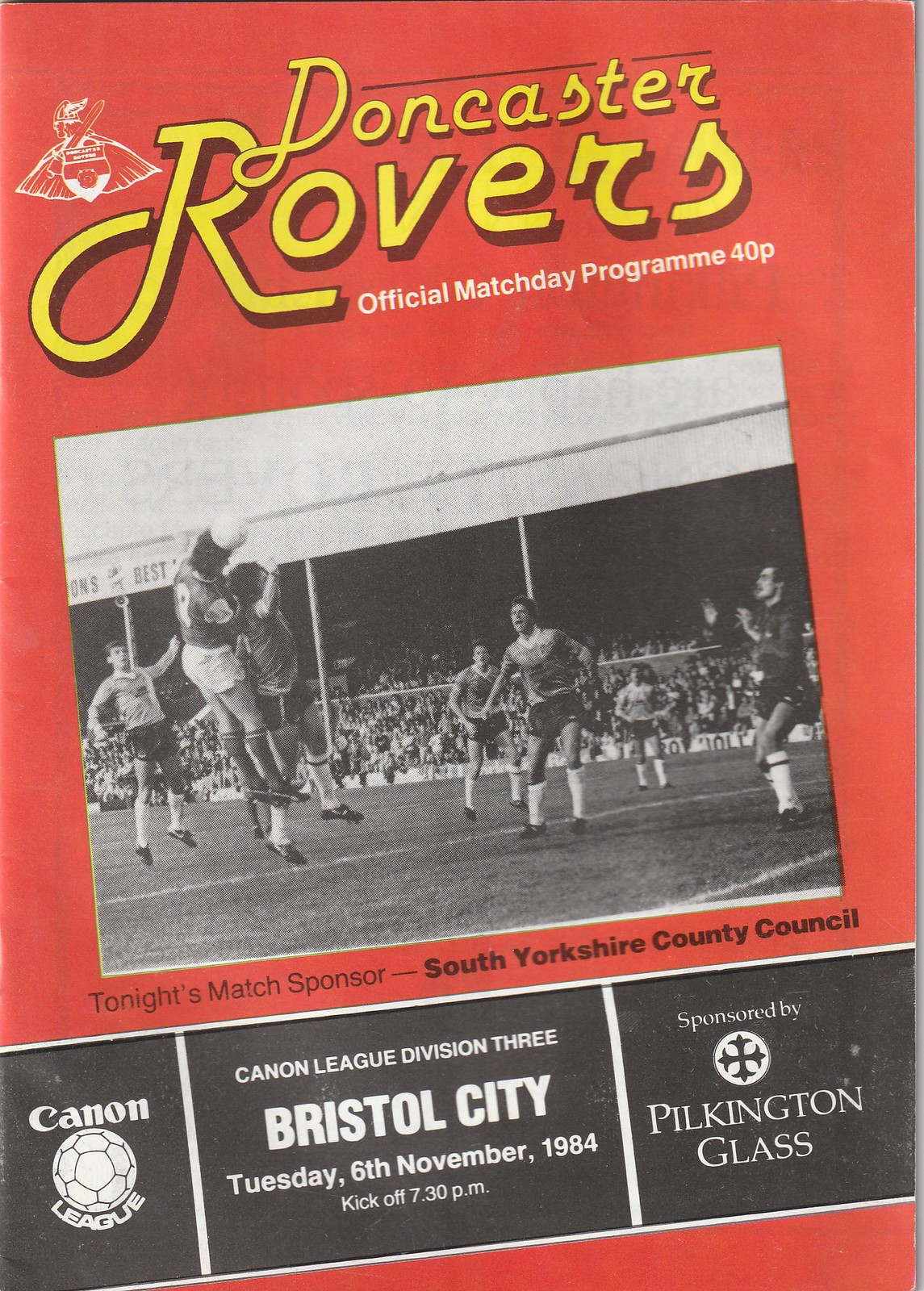This image depicts an official match day program for the Doncaster Rovers football team. The program covers their upcoming game against Bristol City, scheduled for Tuesday, November 6th, 1984, with a kickoff at 7:30 PM. The event is part of the Canon League Division 3 and is sponsored by Pilkington Glass, as well as the South Yorkshire County Council. The program features a red background with "Doncaster Rovers" prominently displayed in yellow. Additional text appears in white or black. The cover includes a black-and-white photo of the players in action, with one player notably leaping to head the ball. The price of the program is listed as 40 pounds. A tagline at the top reads "official match day program."